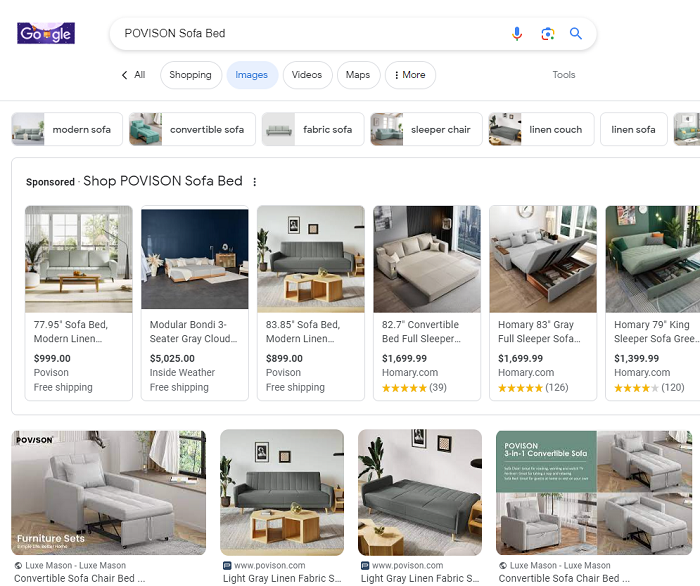Here's a detailed, descriptive caption for the described image:

---
The image illustrates a Google search results page for a "Povison sofa bed." At the very top, the Google icon is prominently displayed in the upper left corner. The search bar below it contains the text "Povison sofa bed." Beneath, the navigation bar shows several tabs including "All," "Shopping," "Images" (which is currently selected), "Videos," "Maps," "More," and "Tools" situated on the far right.

Directly under the navigation bar, there are category buttons for refining the search results: "modern sofa," "convertible sofa," "fabric sofa," "sleeper chair," "linen couch," and "linen sofa." "Fabric sofa" is selected. Below this, the section labeled "Sponsored" appears with the heading "shop Povison sofa bed," displaying a selection of six sofa beds with varying prices.

The listed prices for these sofa beds are as follows: 
- $999
- $5,025
- $899
- $1,099.99 (appears twice)
- $1,399.99

Detailed descriptions of each item are provided:
1. A 77.95-inch modern linen sofa bed from Povison, offering free shipping.
2. A Modula Bondi three-seater in gray cloud from Inside Weather, also with free shipping.
3. An 83.85-inch modern linen sofa bed from Povison, with free shipping.
4. An 82.7-inch convertible full sleeper sofa from Homeree, rated five stars by 39 reviewers.
5. An 83-inch gray full sleeper sofa from Homeree, rated five stars by 126 reviewers.
6. A 79-inch king sleeper sofa in green from Homeree, rated four stars by 120 reviewers.

Below these listings, four additional product images are displayed:
1. A gray convertible sofa chair bed from Povison.
2. A light gray linen fabric sofa, shown in two setups: as a sofa and laid flat as a bed, with a table positioned in front.
3. Another convertible sofa chair bed by Povison, demonstrated in three adjustable positions.

Each of these products is manufactured by Povison, focusing on versatility and modern design.
---

This cleaned-up, detailed caption provides a clear and comprehensive summary of the image and its content.